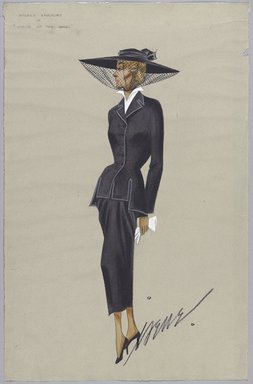This vertical rectangular artwork, likely hand-drawn on light gray paper, depicts a female model in a sophisticated, retro 1950-1960 style. The woman stands facing slightly forward and to the left, with her head turned completely to the left. She wears a large, wide-brimmed black hat adorned with a black veil that completely covers her face and ties around her neck, her short blonde hair subtly visible from underneath. Her attire consists of a black pinstripe, form-fitting blazer over a white collared shirt, paired with a long pencil skirt, black high-heeled shoes, and she holds white gloves or a handkerchief in her left hand, her right arm remaining unseen. The backdrop is a muted gray with some black lines, and the image also contains faint, unreadable text in the upper left corner. A signature, presumably the artist's, is positioned near her feet at the bottom, extending upwards and to the right.